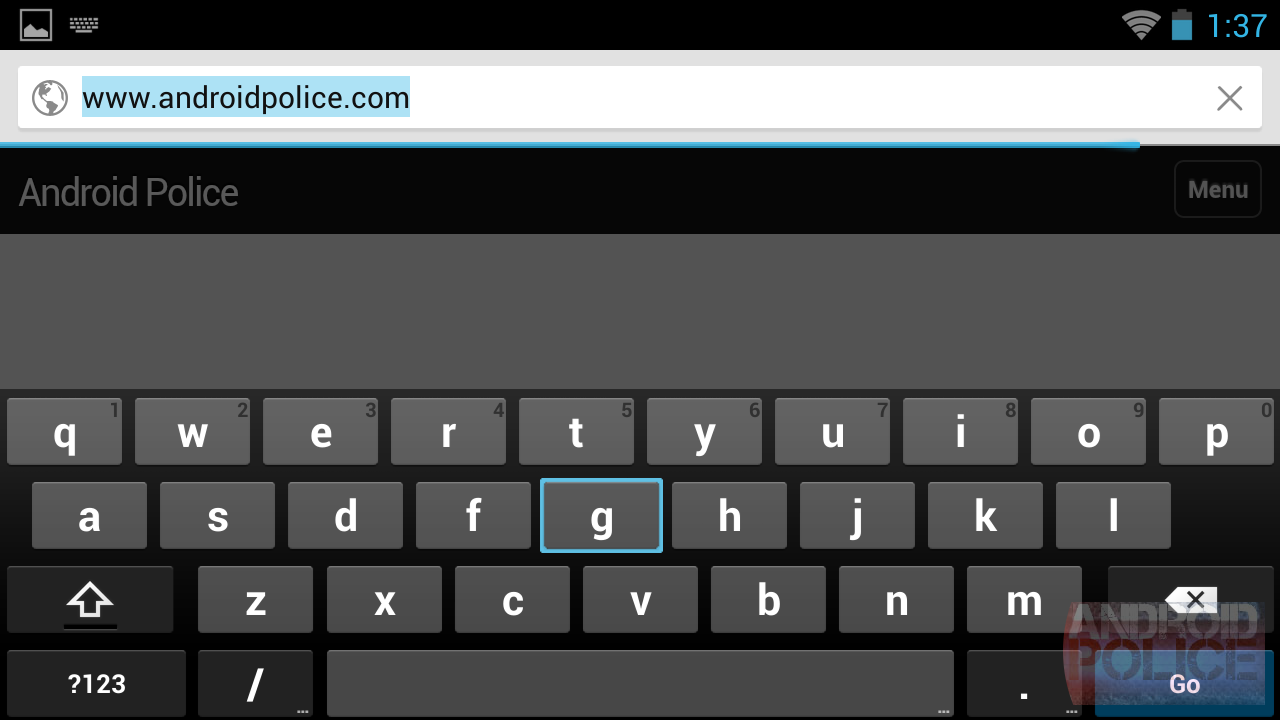The image is a screenshot of a smartphone displaying the Android Police website. At the top of the screen, there is a status bar featuring four icons from left to right: a photo icon, a keyboard icon, a Wi-Fi icon, and a battery icon. The timestamp displayed is 1:37. Below the status bar, there is a globe icon followed by an address bar with the URL "www.androidpolice.com" highlighted inside it. To the right of the address bar is a close (X) button.

Underneath the address bar, the name of the website appears again as "Android Police” in two words, followed by a menu button on the right. The main portion of the image shows the on-screen keyboard, which has gray keys and black function keys. Faintly visible in the background is the website's logo, where the word "Android" is in white and "Police" is in red, housed within a red box. This screenshot captures the interface of a smartphone with the Android Police website open and the on-screen keyboard activated.